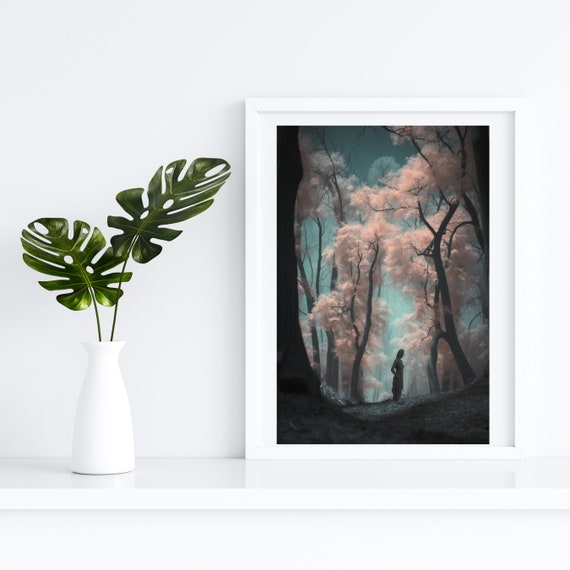The image features a white tabletop against a matching white wall, creating a minimalist backdrop for the items displayed on the table. On the left side of the table, there is an elegantly-shaped white vase with a wider base, a narrow neck, and a flaring mouth. Emerging from the vase are two large, green leaves with distinctive cut-out patterns, including V-shaped cuts and circular holes, supported by long, slender stems. To the right of this vase sits a white picture frame, likely made of plastic or wood, containing a vivid, colorful picture. The image within the frame depicts a forest scene from ground level, capturing a multitude of tall trees with striking foliage that ranges in hues—described variably as yellow, white, or salmon. The sky above the forest is a clear blue, punctuated by white clouds. Central to this forest scene, a shadowed figure of a person stands to the right, while a prominent dark tree trunk occupies the far left foreground of the picture, adding depth to the composition.